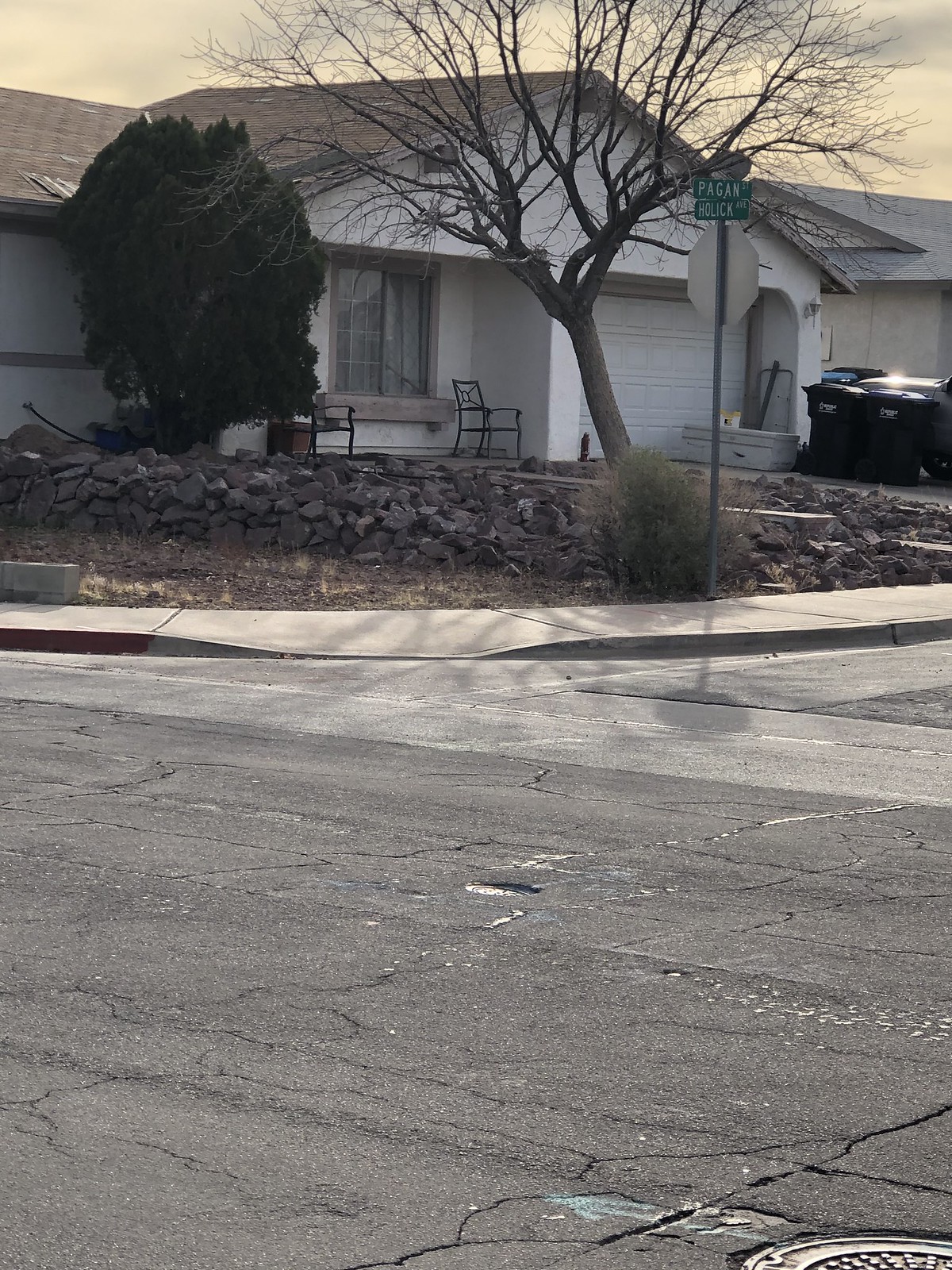In this photo, the viewer is positioned at a street corner, gazing towards the opposite corner. The image captures the rounded edge of a sidewalk that slopes down for accessibility. Prominently in the foreground, the back of a stop sign is visible along with two green road signs indicating "Pagan Street" and "Holic Ave." Beyond these signs, a white house becomes the focal point of the image. The house is situated in a yard filled with rocks. A large, leafless tree stands in the yard, appearing almost lifeless, while a smaller, vibrant green-leaved tree is positioned closer to the front of the house.

Additionally, two chairs are visible on the house's porch area, and the garage door is closed. Outside the garage, there is an object that resembles a tub and several garbage and recycling bins lined up on the front yard area. The overall setting provides a detailed snapshot of a typical suburban corner with a mix of natural elements and everyday objects.